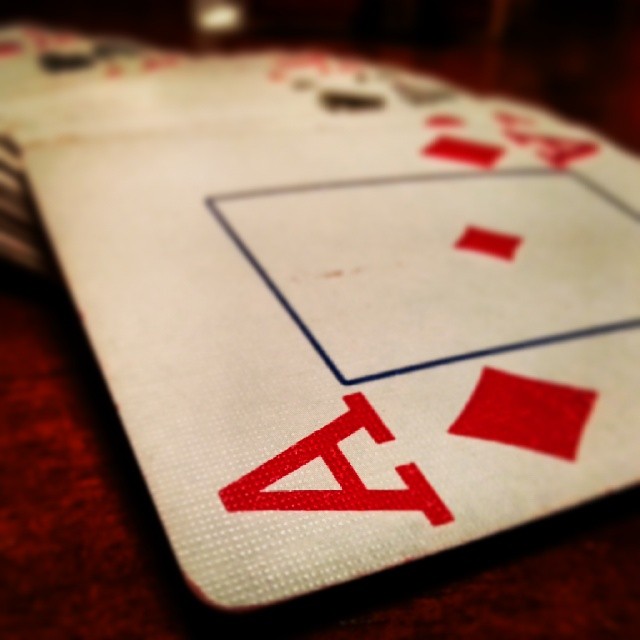This vibrant color snapshot captures an extreme close-up of the Ace of Diamonds playing card. Dominating the foreground, the nearest corner of the card is in sharp focus, revealing intricate details such as its textured, ribbed surface reminiscent of graphing paper with intersecting horizontal and vertical lines creating a dimpled appearance. The edges of the card are notably darker, suggesting either staining or a different dye color along the paper ridge. As the focus recedes towards the far edge of the card, the image becomes increasingly blurred, and the dimly visible playing cards in the background are nearly indistinguishable. The Ace of Diamonds itself is primarily white, featuring a prominent blue rectangle in the center, which encloses a single, vivid diamond icon.